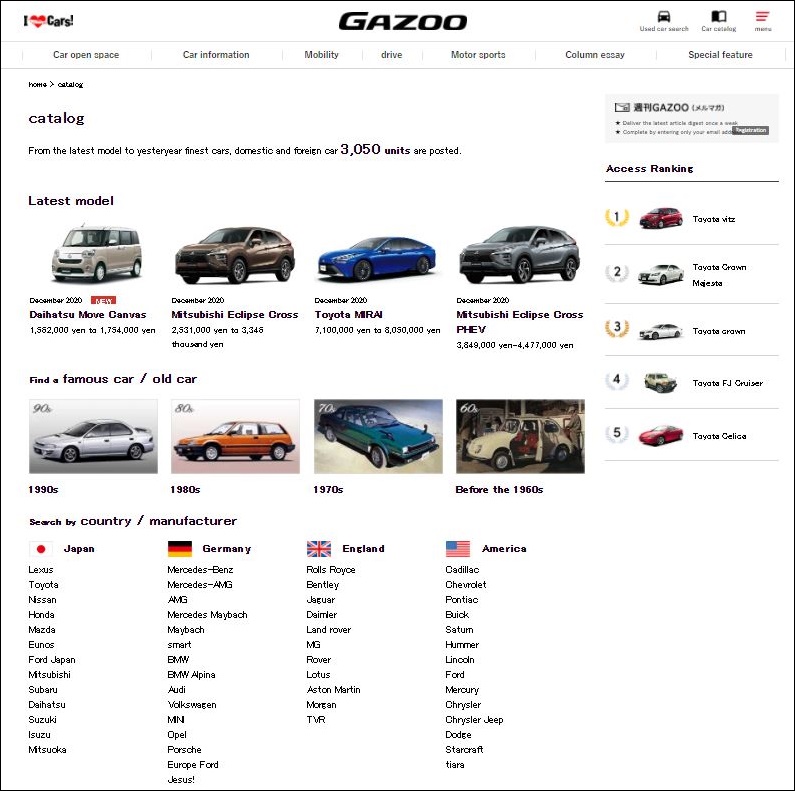In this image, we see a screenshot with a solid white background outlined in gray. In the upper left corner, there is the text "I" followed by a red heart symbol, indicating "I love cars!" Just below this, centered in large black bold text, is the word "Gazoo." In the upper right corner, there is an icon of a car.

Below this header, a menu spans from left to right, consisting of several labeled sections: "Car," "Open Space," "Car Information," "Mobility," "Drive," "Motorsports," "Column," and "Special Feature."

On the left side, below the menu, there is bold text reading "Catalog." Below this heading, the latest models are displayed, starting with a row of four car images. From left to right, these images feature:
1. A small silver car.
2. A Mitsubishi Eclipse crossover.
3. A blue Toyota car.
4. Another silver Mitsubishi Eclipse cross.